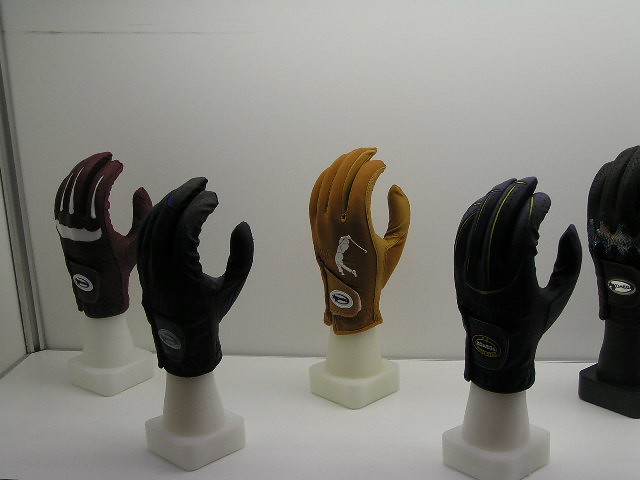In a brightly-lit white display case, a collection of golf gloves is meticulously arranged on white stands that give each glove a lifelike appearance as if worn on a hand. These leather gloves, designed with both functionality and style in mind, feature various colors and details. From left to right: a distinctive dark brown glove is followed by a light brown tan glove that prominently displays a white image of a golfer, emphasizing its sporty purpose. Next, a sleek black glove stands out, completely black in color. Further along, there is an eye-catching orange mustard-colored glove, and to its right, a glove with striking yellow lines adding a pop of color. Lastly, another black glove catches the light, this time enhanced with mesh detailing for added texture and breathability. Each glove is adorned with a medallion on the wrist, reflecting the sophisticated branding. The display is carefully illuminated from above, highlighting the craftsmanship and detail of each glove.